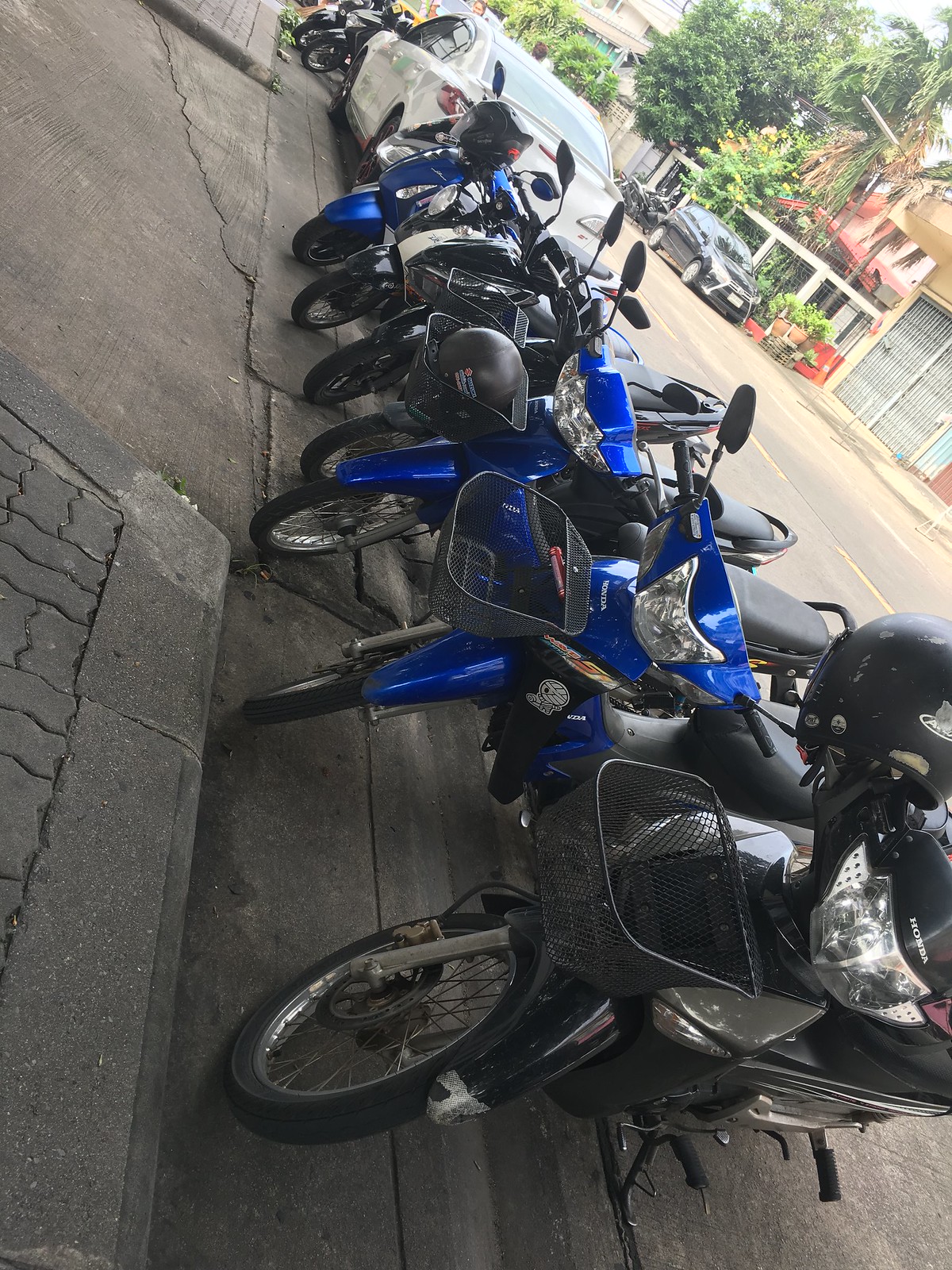This photograph features a row of motor scooters parked perpendicularly to the curb on a cracked city sidewalk. The scooters, which appear to be mopeds, are predominantly black and blue, with at least three of them sporting helmets hanging from their handlebars or baskets. Notably, some of these scooters are Hondas, easily identified by their logos. A white Mazda 3 is parked parallel to the street behind the scooters, partially dividing the line of mopeds. In the background, a compact black car is visible across the street, alongside buildings and houses partially obscured by trees and plants. The image is taken at an unusual angle, adding a disorienting effect, with the row of scooters extending from the bottom right to the top center of the image, framed by the gritty urban environment.